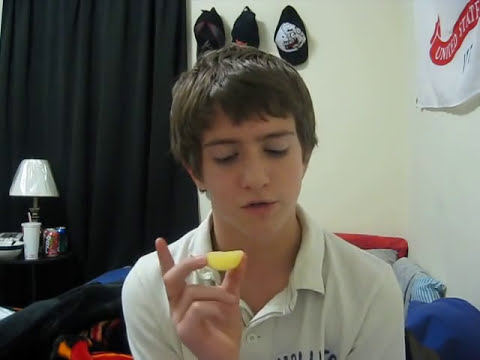In this detailed image, a boy aged around 10 to 14 years, dressed in a white collared polo shirt, sits upright on the edge of his bed in his bedroom. His short, shaggy brown hair slightly covers his forehead but does not reach his ears. The boy is intensely focused on a lemon wedge held delicately between his thumb and middle finger, with his index finger pointing up and his other fingers tucked in. 

The bedroom backdrop includes a variety of items that give it a lived-in feel. Behind him, a red-framed bed is adorned with a mix of colorful blankets in shades of red, black, and blue, alongside a blue and white striped pillow. The white wall behind him features three hats hanging in a neat row: one is red and black, another is white and black, and the third is entirely black. Adjacent to these hats is a fabric banner declaring "United States" in white letters on a red ribbon background, set against a larger white cloth.

To the right of the scene stands a nightstand with a white lamp, still wrapped in plastic, and topped with a white shade. Underneath the nightstand, there are cans of soda, including a red Mr. Pibb can and what appears to be a Sprite can, along with a white cup and a bowl. To the left, a black curtain or shade adds a dark contrast to the otherwise light-filled room. The overall setting is clearly his bedroom, capturing a quiet moment of the boy examining the lemon wedge in his hand.